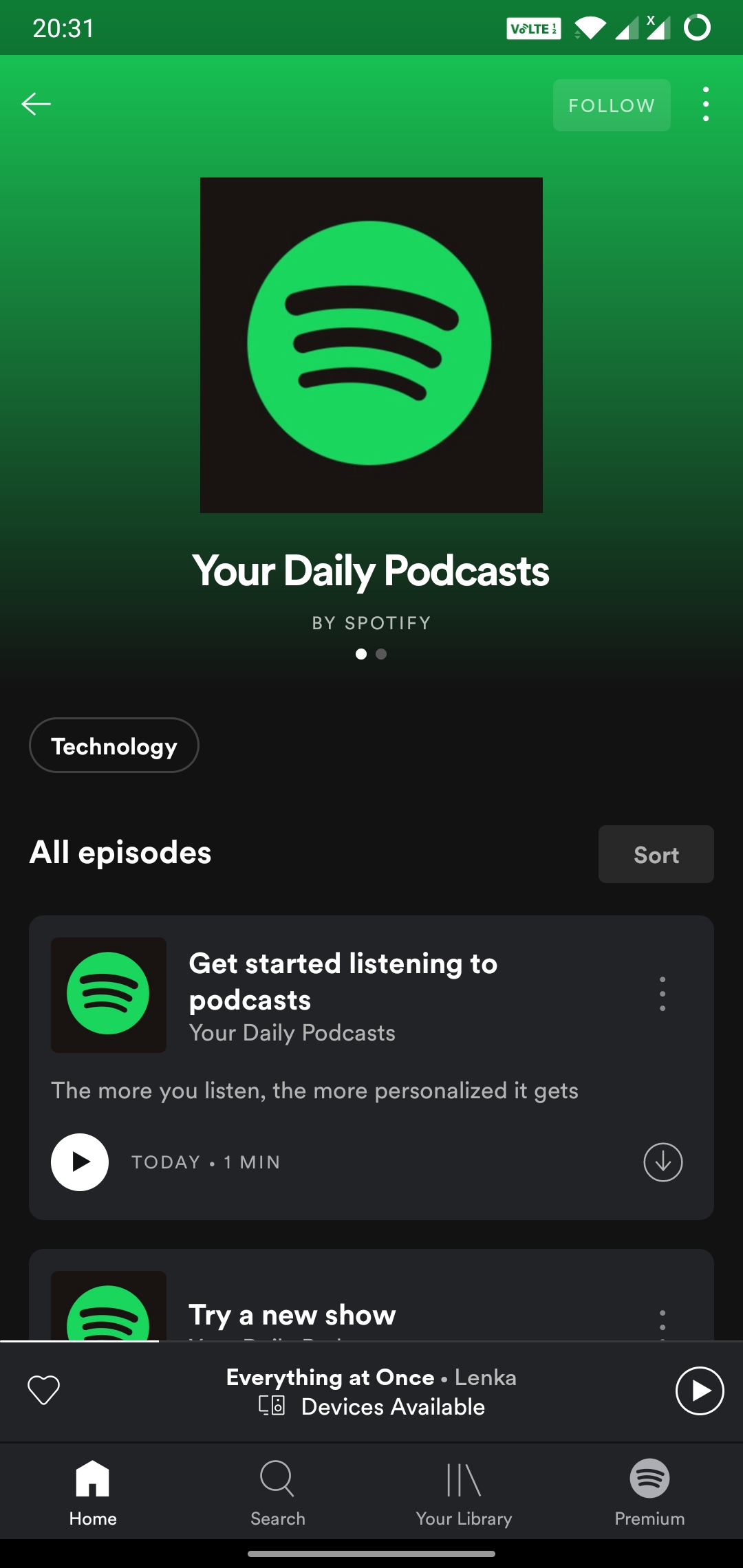This is a screenshot from the Spotify mobile app. At the top of the image, the status bar displays the current time as 20:31. In the upper right corner, there is a small white rectangle with the text "WLTE" in green, indicating the carrier. Next to it, the Wi-Fi icon shows a full signal, while the mobile signal is at half strength. A small white circle is also visible in the status bar, possibly indicating a notification.

Below the status bar, the Spotify interface is open, featuring the iconic Spotify logo—a black square with a green circle in the center, containing three black horizontal slashes. Beneath the logo, white text reads "Your Daily Podcasts by Spotify," flanked by two white dots. Further down, an outlined oval with "Technology" written in white font is visible, signifying the category. Underneath this, the words "All Episodes" appear in white font, with a small gray rectangle labeled "Short" in white font beside it. The section below lists episodes, which appear to be tutorials on how to listen to podcasts.